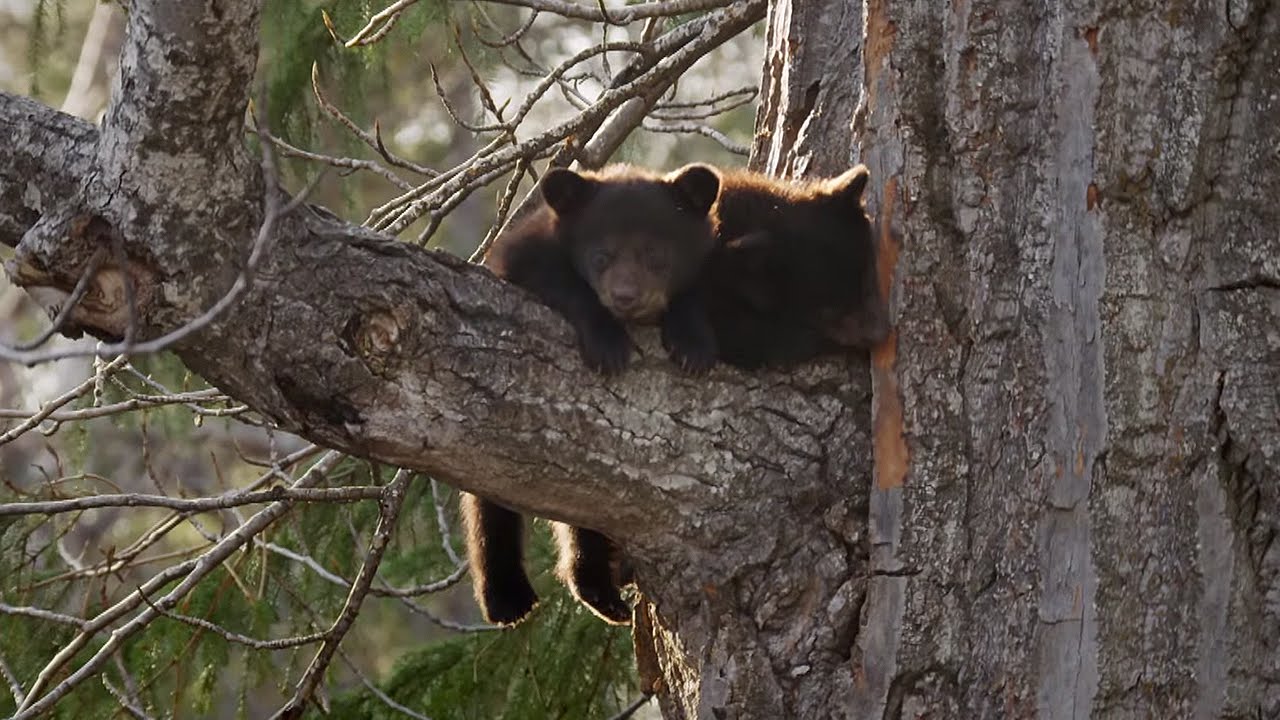This is a horizontally aligned, rectangular close-up photograph capturing an outdoor scene featuring two baby brown bear cubs clinging to a thick tree branch. The large tree trunk occupies the right side of the image, with parts of its bark peeling and the trunk extending beyond the frame both above and below. One thick branch emerges from the middle of the trunk, extending diagonally toward the upper left corner, and is adorned with numerous smaller branches.

The two cubs are located where this thick branch meets the tree trunk. The cub on the right appears to be gnawing on the tree bark, and only its head, ears, and part of its chest are visible. In contrast, the cub on the left looks directly towards the camera with its ears perked up, appearing more fully suspended from the branch, with its feet dangling below. Both cubs have lighter brown snouts and fluffy ears.

Behind the bears, the background is filled with green foliage and thinner tree branches, somewhat out of focus, highlighting the depth of field in the photograph. The sunlight streams in from the top left, illuminating the backs of the bear cubs, suggesting it is daytime.